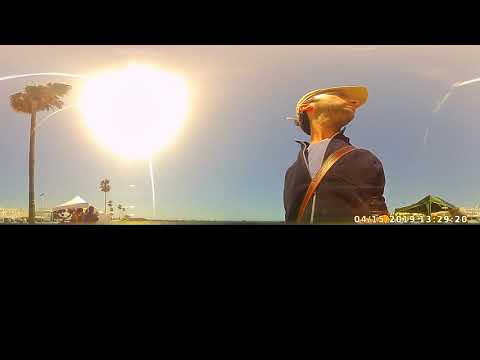The photograph depicts an outdoor scene dominated by a vibrant sky stretching overhead. This panorama is unusually wide compared to its height, with a significant black band obscuring the lower third of the image featuring a yellow time and date stamp. Central to the composition is a man, seen from a low angle, creating an upward gaze. He's wearing a light gray or blue t-shirt beneath a dark zippered jacket, complemented by a leather strap draped across his left shoulder. A baseball cap, possibly white or yellow, shades his face, and his dark hair is visible underneath, along with the cap's adjusting strap at the back.

The man appears to be glancing behind him, seemingly alert or cautious. Sunlight bursts brightly from the left side of the image, casting a glare that suggests late afternoon or early morning. A tall palm tree anchors the left edge of the photo, near a white canopy or tent. To the right, another green canopy is situated, set against streaks of white clouds in an otherwise blue and gray overcast sky, adding a hint of an ominous feeling. Adding to the scene's open-air ambiance, the expansive landscape stretches towards the horizon, indicating a spacious, perhaps beachside or recreational setting.